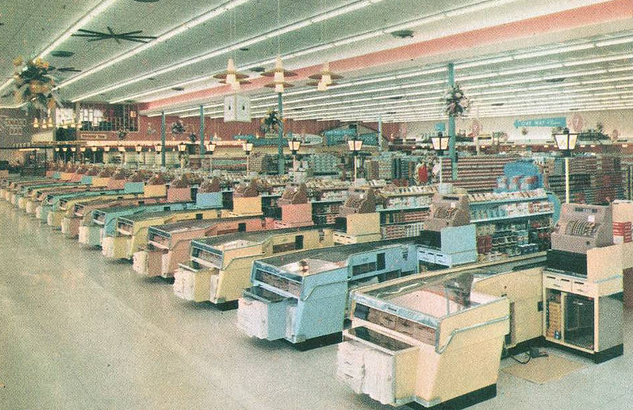The image depicts a vintage grocery store, most likely from the 1960s or 1970s, with an expansive view of numerous checkout lanes arranged in a neat, colorful sequence. The photo, rectangular in shape, shows the tops and bottoms as the longer sides. The checkouts start from the bottom right and extend to the left, disappearing into the distance. The counters display a vibrant palette in a somewhat alternating pattern: yellow, blue, yellow, red, and repeat. Each counter is equipped with an old cash register, a conveyor belt to the left, and bins beneath, possibly holding bags. A little cabinet with glass doors is visible under the register at the closest checkout.

Above, a gray ceiling adorned with black decals, ceiling fans, and lights spans the length of the store, creating a uniform look. There's also a hanging plant and a message box positioned around the left-middle area of the ceiling. The white tiled floor complements the color scheme of the counters, and on the right side of the checkouts, grocery aisles stretch into the distance. Far-off windows allow natural light to filter in, adding to the inviting ambiance of this retro setting.